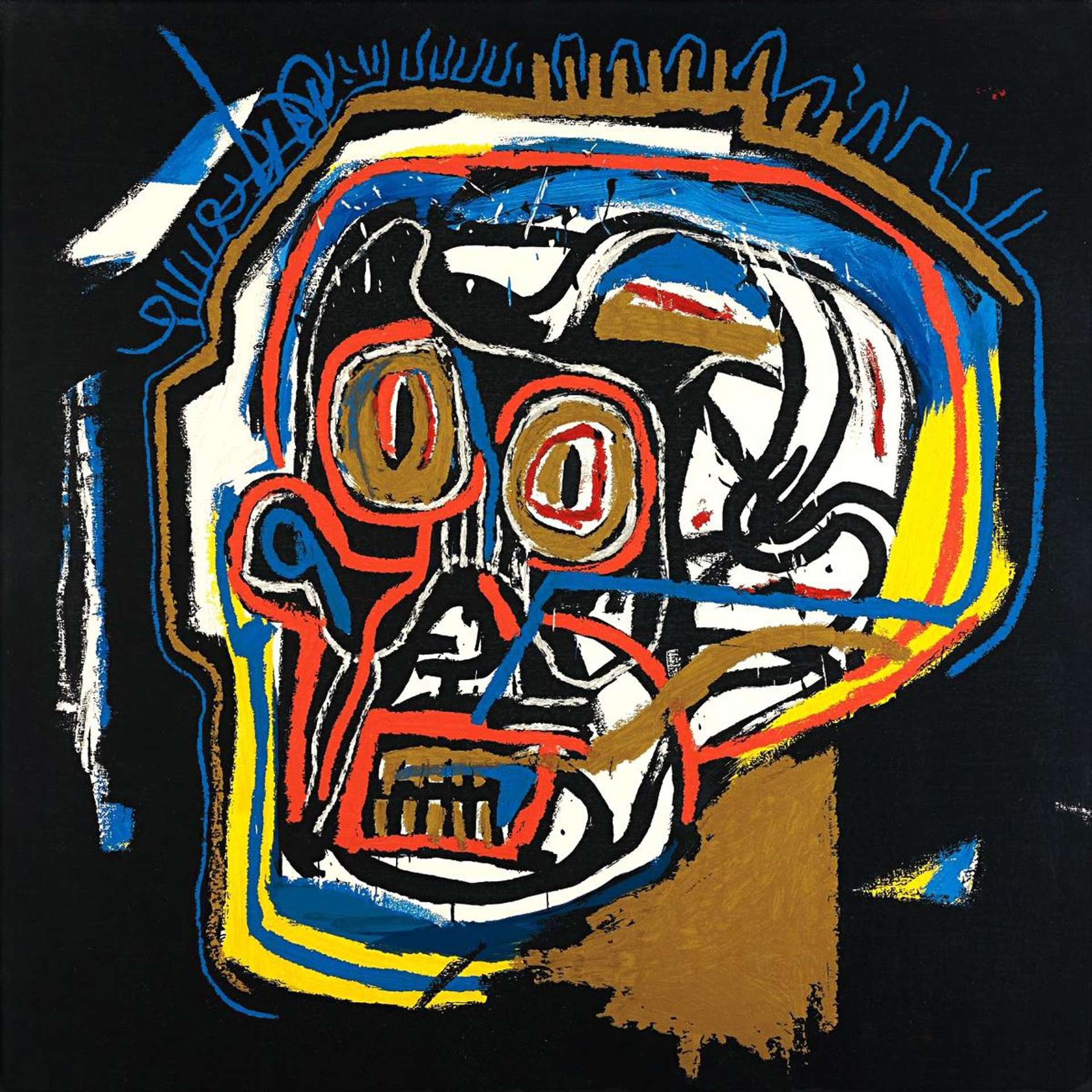The image depicts a piece of modern art featuring a human skull superimposed on a black background. The skull, predominantly white, has a mixture of striking colors and intricate details. The eyes are circled with concentric rings of red, brown, white, and orange. The teeth are outlined in white with brown highlights. The artwork is adorned with blue squiggly lines at the top, which extend to the left border. A brown border also runs from the top of the skull down the left side. Additionally, there is an orange border around the skull itself, interspersed with blue and yellow accents. Notable elements include white stripes infused with blue at the crown of the skull and a triangular section on the right side displaying yellow and blue hues. The details such as the lips, hairline, and facial features, along with the color palette of brown, blue, yellow, red, and black, contribute to the eerie and intriguing aesthetic of this painting.